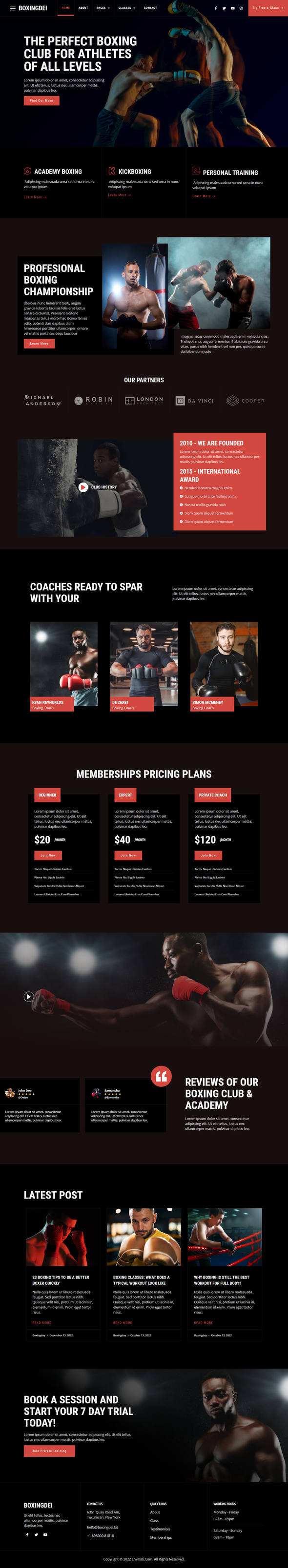This screenshot features an advertisement or promotional content with a solid black background, though it is slightly blurry. In the upper left corner, the website name appears to start with "boxing" followed by indistinct letters that could be "D," "DEI," or "DE1." In the upper right corner, there is a noticeable red box containing the word "class." Dominating the top section of the image, two men in dark shorts are depicted in a boxing match; the man on the left is mid-action, throwing a punch towards the abdomen of the man on the right. To the left of this boxing scene, bold white text reads: "The perfect boxing club for athletes of all levels." Directly below that is another line of white text stating: "Professional Boxing Championship." Towards the bottom left of the image, another line of white text encourages action with: "Book a session and start your seven-day trial today." To the right of this text, a young black man is shown from the chest up, looking forward confidently without a shirt.